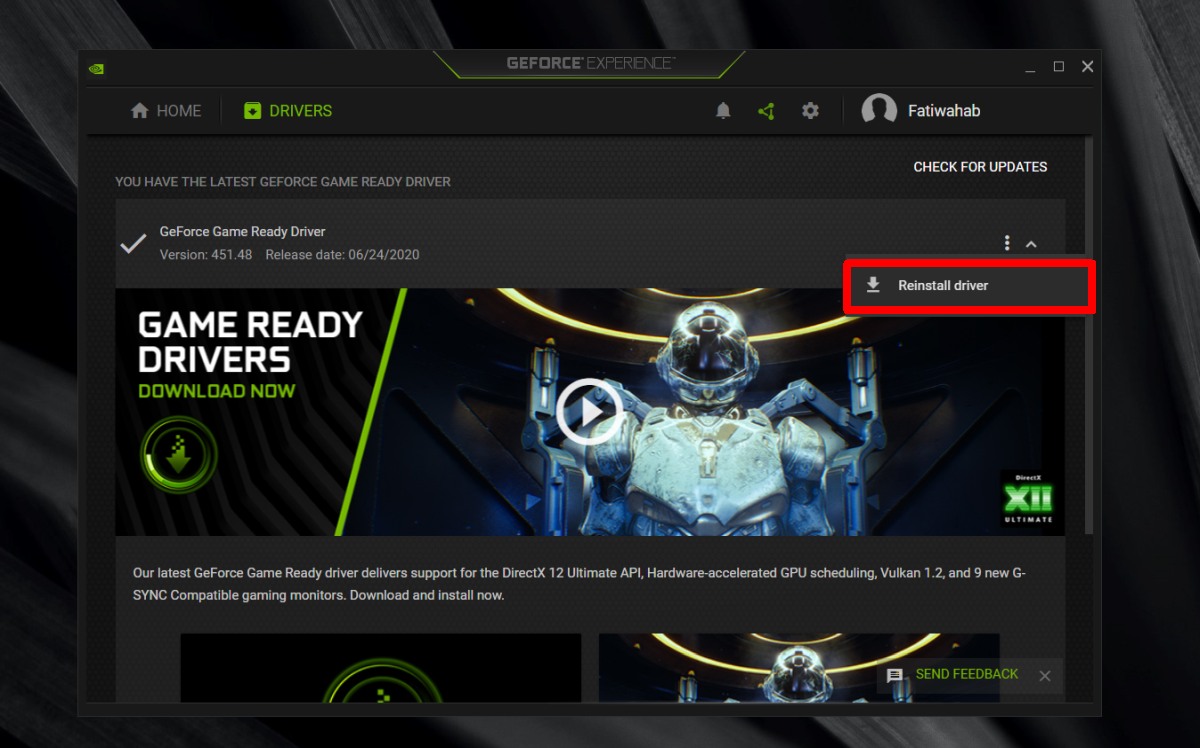In the image, a GeForce Experience interface is displayed against a stark black background. At the very top center, "GeForce Experience" is prominently featured, encased in a sleek green outline. In the top left corner, there is a small green icon. Below, notable interface elements include a black "Home" button, followed by a green "Drivers" button, accompanied by several other smaller icons. 

On the top right, there's a circular profile picture of a person labeled "Fatty Wayhab," alongside the typical window control buttons: a square for maximizing, an 'X' for closing, and a dash for minimizing. Just beneath these, the text "Check for updates" indicates the feature's availability, stating that "You have the latest GeForce Game Ready Driver" with a corresponding checkmark for confirmation. It specifies the driver version and release date next to this statement.

Further down, highlighted against the black background, "Game Ready Drivers Download Now" stands out in vibrant green text. Beneath this, a vivid image of a sci-fi astronaut is shown. A white circle with a right-facing arrow is superimposed over this image. Adjacent to this imagery, there is a gray box outlined in red featuring a down arrow and the text "Reinstall Driver."

In the lower right corner of the image, "X11" is showcased in green text within a black box. The caption below describes, "Our latest GeForce Game Ready Driver delivers support for the DirectX 12 Ultimate API, hardware-accelerated GPU scheduling, Vulkan 1.2, and 9 new G-Sync compatible gaming monitors. Download and install now."

Lastly, at the very bottom, there are two additional images, and prominently positioned near them is a button labeled "Send Feedback."